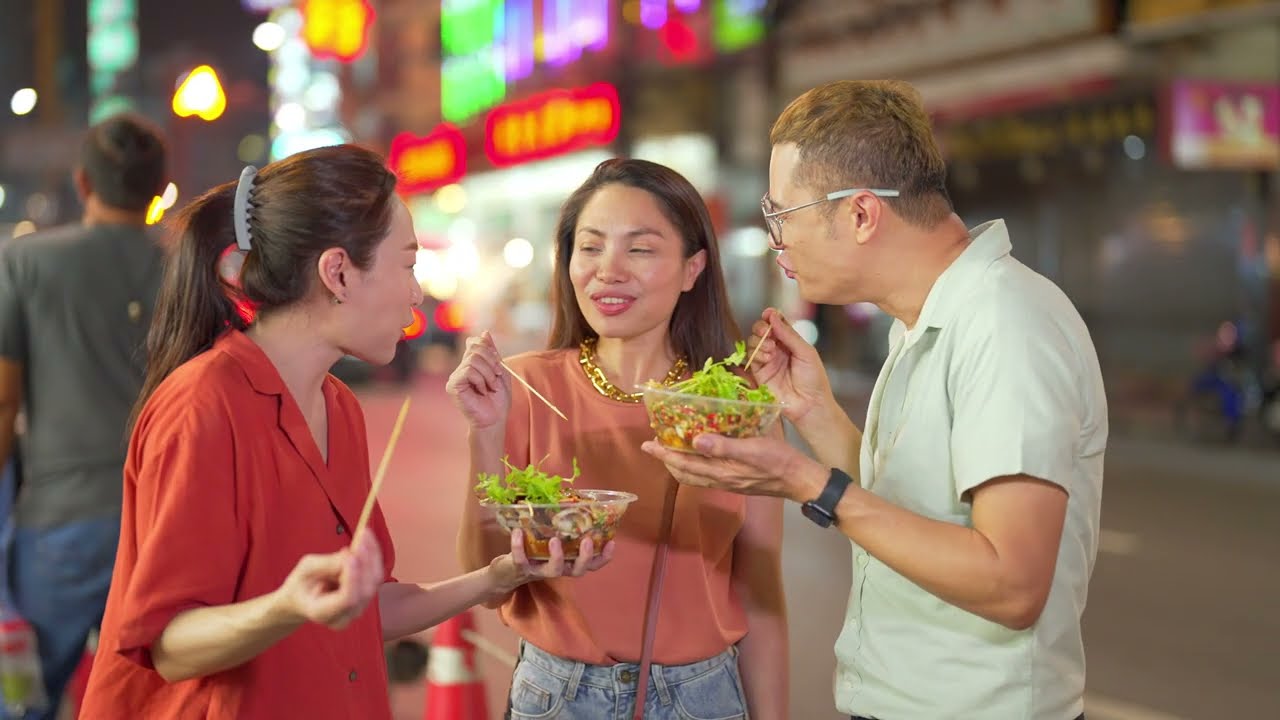In an evening cityscape, three people of Asian descent are enjoying a meal on a bustling sidewalk filled with neon lights, blurred storefronts, and passing pedestrians. In the foreground, two women and a man stand eating with chopsticks while sharing two bowls of food featuring leafy green vegetables and other indistinct ingredients. The woman on the left is dressed in a red collared button-up shirt, her hair pulled back with a clip, holding a bowl in her left hand and chopsticks in her right. The woman in the middle, wearing a peach-colored top, blue jeans, and a gold necklace, has long brown hair cascading down her back. Her left hand rests by her side while her right extends a chopstick towards the bowl held by the woman on the left. The man on the right, sporting a white short-sleeved shirt, a black watch, and glasses, holds a bowl in his left hand and uses chopsticks with his right. The background reveals a lively city street adorned with various neon signs and bustling activity, creating a vibrant and energetic atmosphere typical of an urban evening.